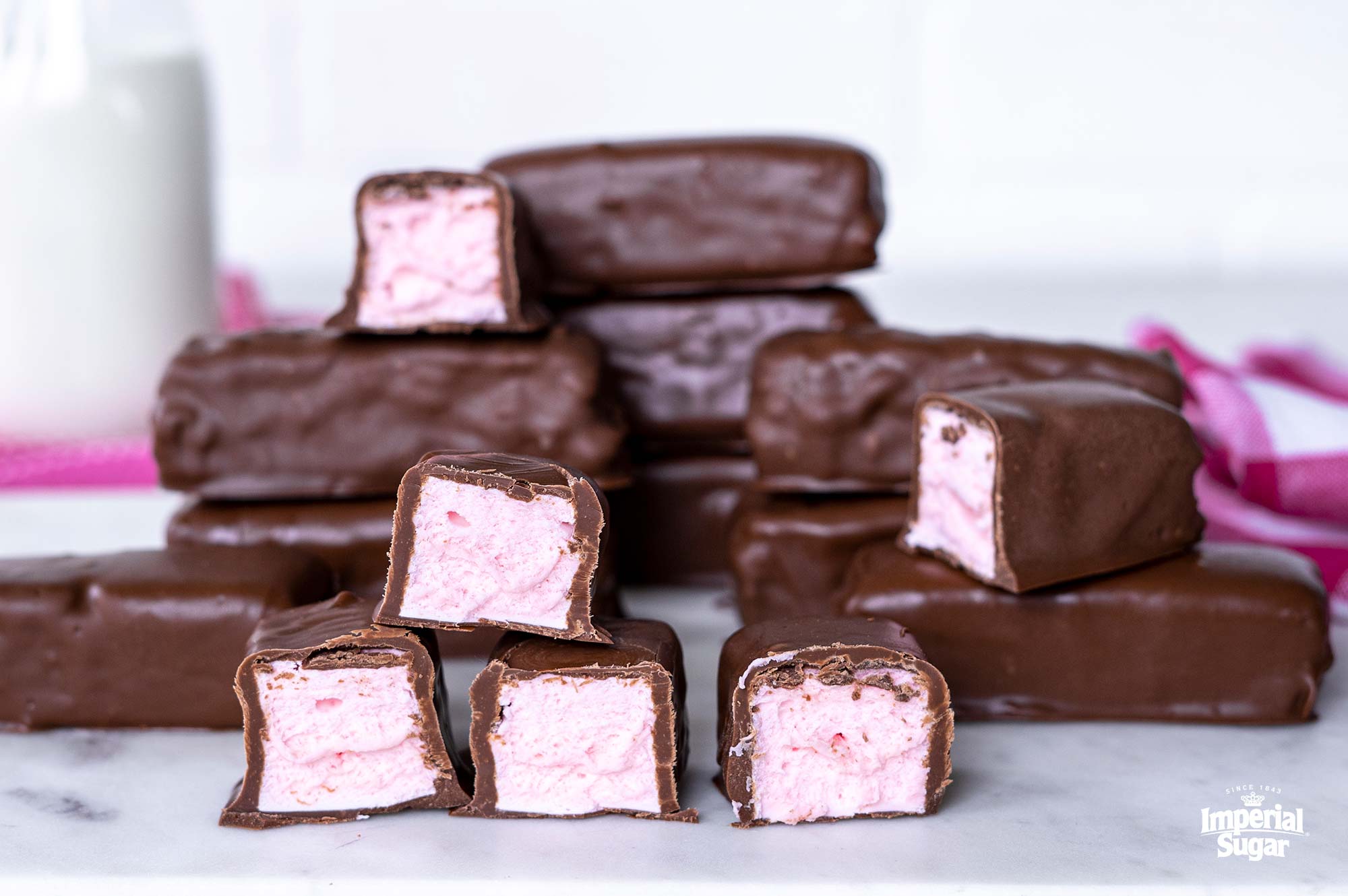This photograph features an assortment of chocolate-covered candies, prominently displayed on a flat surface. The image showcases three pairs of halved candies at the forefront, exposing their dense, pale off-white nougat filling. Behind these are stacks of nine additional candy bars in their entirety, all coated in a thin layer of lush brown milk chocolate. The rectangular bars resemble mini snack or dessert treats, akin to the shape of a Snickers bar. Adding a touch of color, a pink cloth napkin is situated in the middle right side of the image. Notably, the word "imperial sugar" can be seen in the lower right corner. This detailed arrangement paints a vivid picture of delectable, chocolate-coated confections, inviting and appetizing to any viewer.